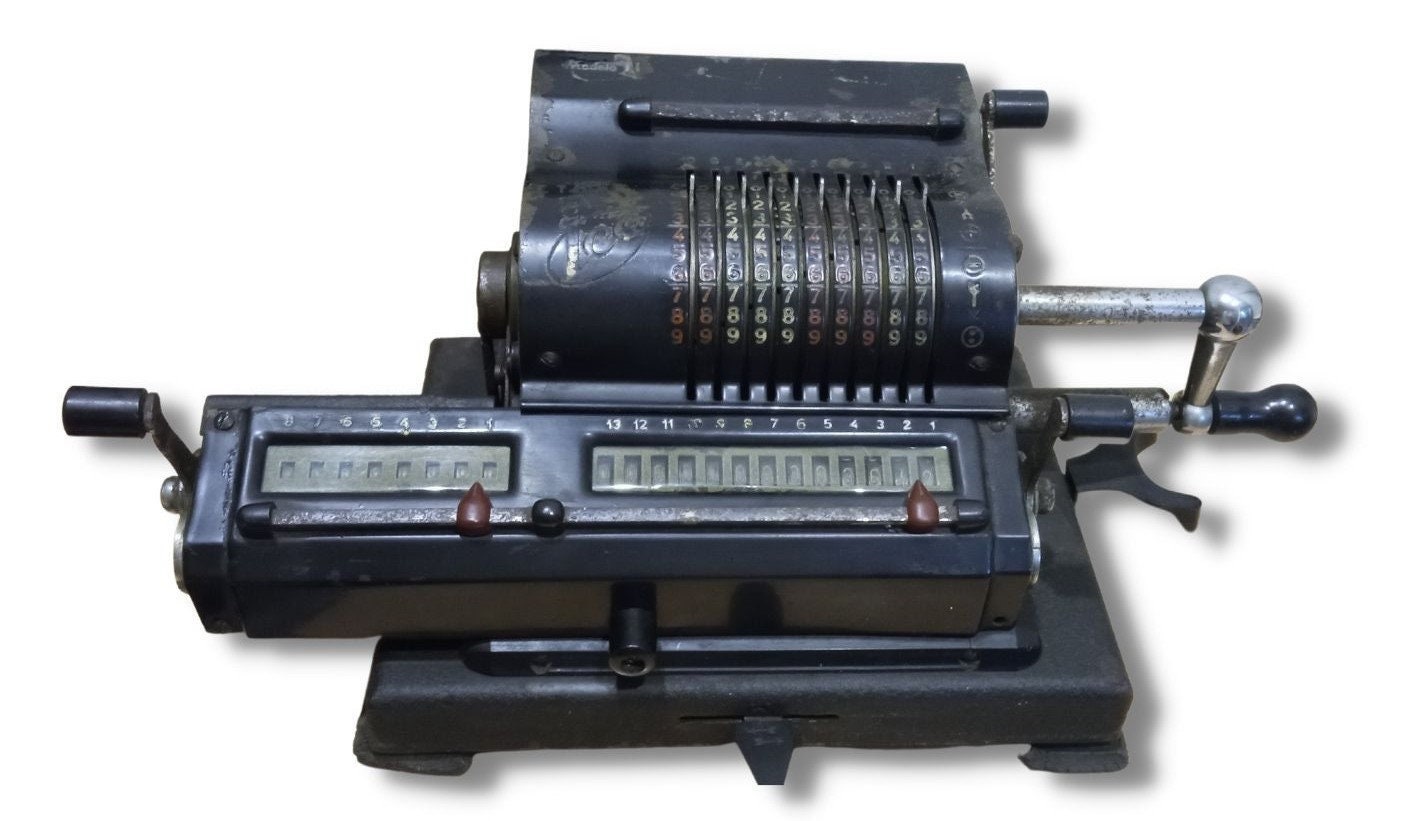This image depicts an antique black metal calculating machine resting on a white background. The machine features a cylindrical top portion equipped with a crank handle, which is used to rotate the numerical values displayed. Below this, the device boasts multiple rows of numbers, each ranging from 1 to 9, with small latches above each number that can be manipulated to set the desired figure. The machine also includes several additional crank handles, emphasizing its manual operation. The lower section appears to house a box-like compartment, possibly for storing cash or collected data, adding to the machine's functionality. Although some parts are worn or scratched, the intricate details of the handles, sliders, and numeric settings indicate this is a sophisticated mechanical calculator, likely predating electronic versions.